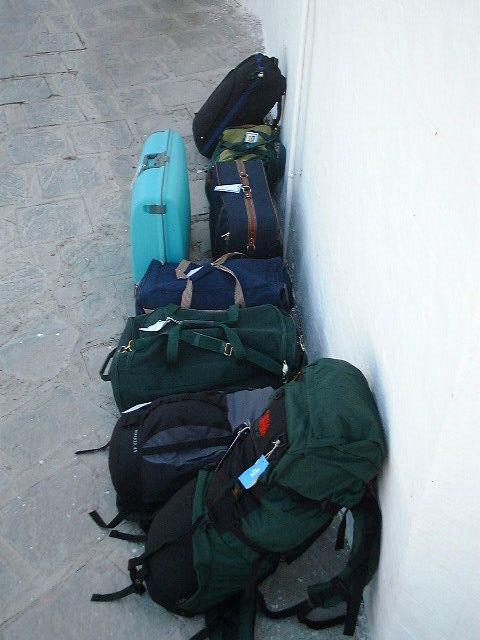The image is a top-down, vertical photograph showcasing eight pieces of luggage neatly arranged against a white wall on the right side, possibly exterior. The floor is a dark brownish-gray, brick-paved sidewalk. The foreground features a large green backpacker's rucksack standing upright, all pieces with temporary tags likely from an airport or train station. Next to the rucksack lies a smaller backpack on its side, followed by a large gray and black backpack. There's a green duffel bag with regular handle straps and an over-the-shoulder strap, and a blue duffel bag as well. Behind these lies a vintage-style, hard-sided aqua blue suitcase standing upright, and a similarly positioned soft-sided blue suitcase with leatherette trim. Partially hidden is another small green backpack, and finally, there's a black rolling soft-sided suitcase. The overall scene depicts various travel bags, mostly dark in color, arranged in an orderly manner, capturing a transient moment of travel preparation or arrival.